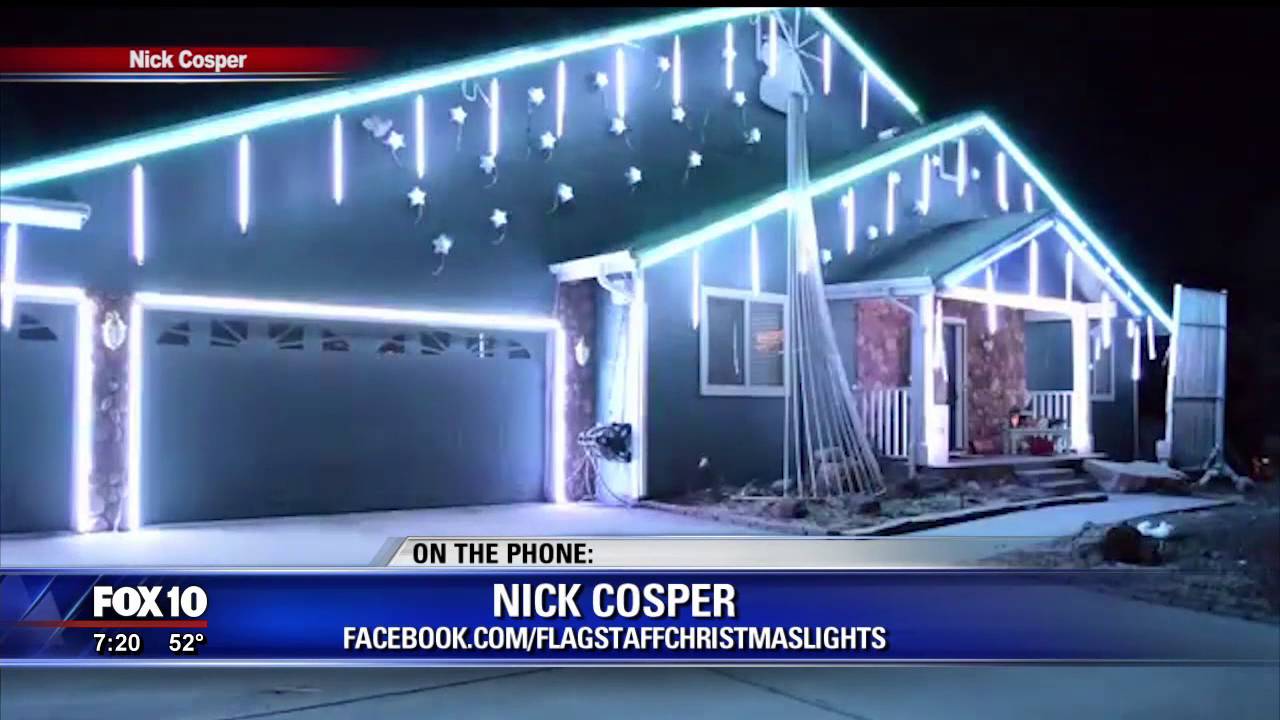This photo is a screenshot from a Fox News affiliate broadcast featuring an extensively decorated house for Christmas. The house, attributed to Nick Kosper via a red insert with his name in white writing in the top left corner, showcases an elaborate display of bluish-green LED and white lights. The bottom left corner of the image displays a Fox 10 banner indicating a temperature of 52 degrees and a time of 7:20. The banner also promotes a Facebook page, facebook.com/FlagstaffChristmasLights, associated with the homeowner.

The house itself is predominantly visible on the right side of the image, with the left side shrouded in night darkness. It features a triangular, slanted roof adorned with icicle lights and a large snowflake in the front, complemented by smaller steeples also garnished with icicles and bluish-green lights. The garage door is framed by white lights and the one-car garage visible is partially in view. The entrance porch, accessible by four steps lined with white gates, is similarly decorated, with stonework around the door illuminated.

A notable feature in the front yard is a large, metal-like tree structure topped with a star. The ground appears to be snow-covered, enhancing the wintry ambiance of this picturesque Christmas scene.